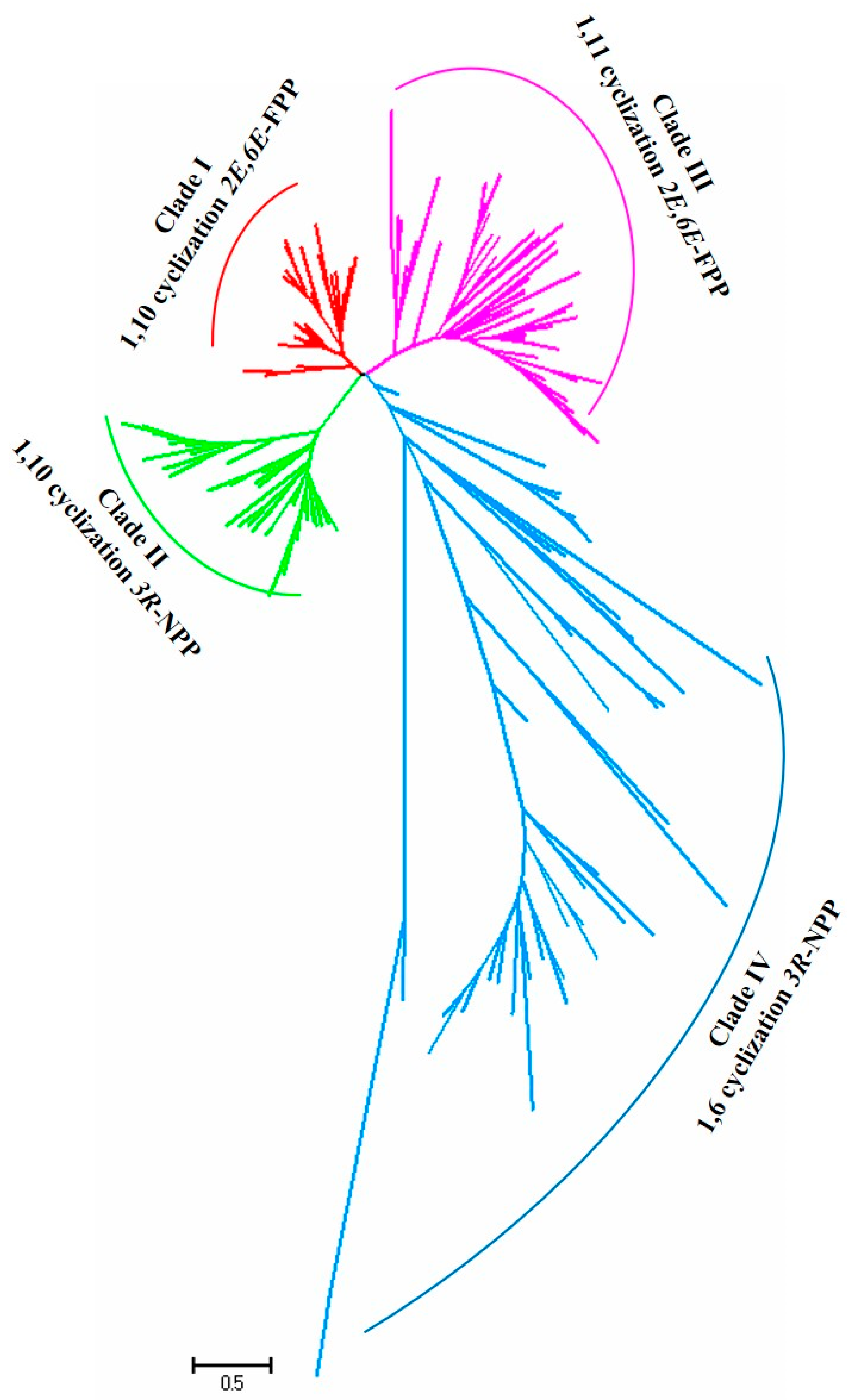The image is a detailed, multicolored diagram consisting of branching lines emanating from a central focal point, resembling tree branches with varying lengths and structures. The lines are color-coded with red, green, blue, and pink hues representing different clades, specifically labeled as clade I, clade II, clade III, and clade IV in Roman numerals. These labels are accompanied by detailed measurements such as "1.10 cyclization" and "1.60 cyclization," indicating some form of structural or numerical data. Across the top of each clade, the branches are capped by a semicircle or conical shape in the respective color. The red lines of clade I are smaller and more condensed, the green lines of clade II are somewhat larger, the pink lines of clade III are even larger, with the blue lines of clade IV being the most extensive and complex. Each clade’s branches are interconnected at their bases, and the diagram is annotated with black text on a white background, providing further descriptions beneath each clade number.